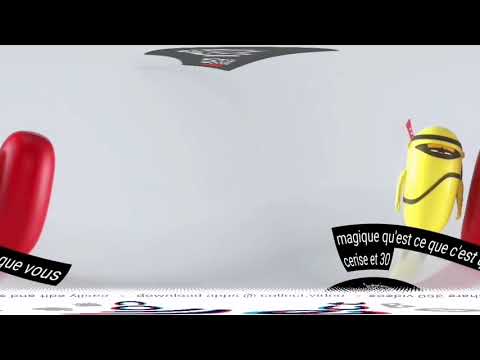In this image, we see a drawing with a light gray off-white background framed by thick black borders along the top and bottom. The image features two distinct capsule-shaped objects positioned on opposite sides. On the left, there is a glossy red 3D capsule tilted diagonally, while on the right, a yellow capsule, resembling a fingernail with faint eyes and thin arms, stands upright. Both capsules have small visor-like details on them.

Text in white letters on black banners is spread across the image. Directly below the yellow capsule, the text reads "MAGIC-CASSE-CULTURE-SERIES-EFFERTY," appearing to be French. Further details include "MAGIQUE QUEST, C-E Q-U-E C-E-S-T, CERISE 30." On the left side, underneath the red capsule, is the text "QUEVOUS." The bottom of the image features another white banner with unreadable text, possibly also in French. There is some small overlay text at the very top of the screen, and another dark gray object of indistinguishable form above one of the black borders. This drawing appears to be a piece of digital art, possibly shared on social media.